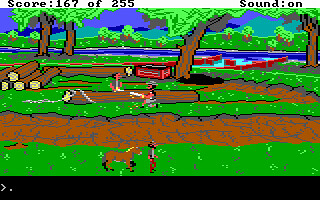This is a screen capture of a computer game in progress featuring pixelated and basic graphics. The scene depicts a forest being cut down, with a narrow road running horizontally across the image. In the foreground, a man stands with his horse adjacent to the road. Across from them, two men are engaged in sawing a log; both grasp the ends of a large saw. Behind these men is a neat stack of logs already processed. Nearby, there is a brown and red box. The background features some standing trees amidst lush greenery, with a river flowing horizontally beyond the trees. Further behind, the landscape transitions into rolling green hills and distant mountains under a clear sky.